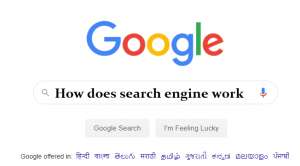This image is a vertical screenshot of the Google search engine, potentially captured in India, indicated by the presence of language cues. At the top of the image is the colorful Google logo, featuring a blue capital 'G', a red 'O', a yellow 'O', a blue lowercase 'g', a green 'l', and a red 'e'. Directly below the logo is an elongated search bar with rounded edges, reminiscent of a long vitamin pill in shape. Within this search bar, the black, bold text reads "How does search engine work," with the 'H' in "How" capitalized and no punctuation.

Inside the search bar, to the left of the text, is a search icon, and to the right is a microphone icon adorned in Google's characteristic colors: a blue microphone with a reddish-yellow arch and a touch of green at the base. Below the search bar, two grey buttons are placed side by side; the left button displays "Google Search," and the right button says "I'm Feeling Lucky."

Further down, the text "Google offered in" is visible, followed by an array of blue hyperlinks in a script that appears to be Hindi or a similar language, suggesting the localized nature of the search engine's interface. The background, blending into surrounding elements, makes it slightly challenging to identify the exact top and bottom of the image.